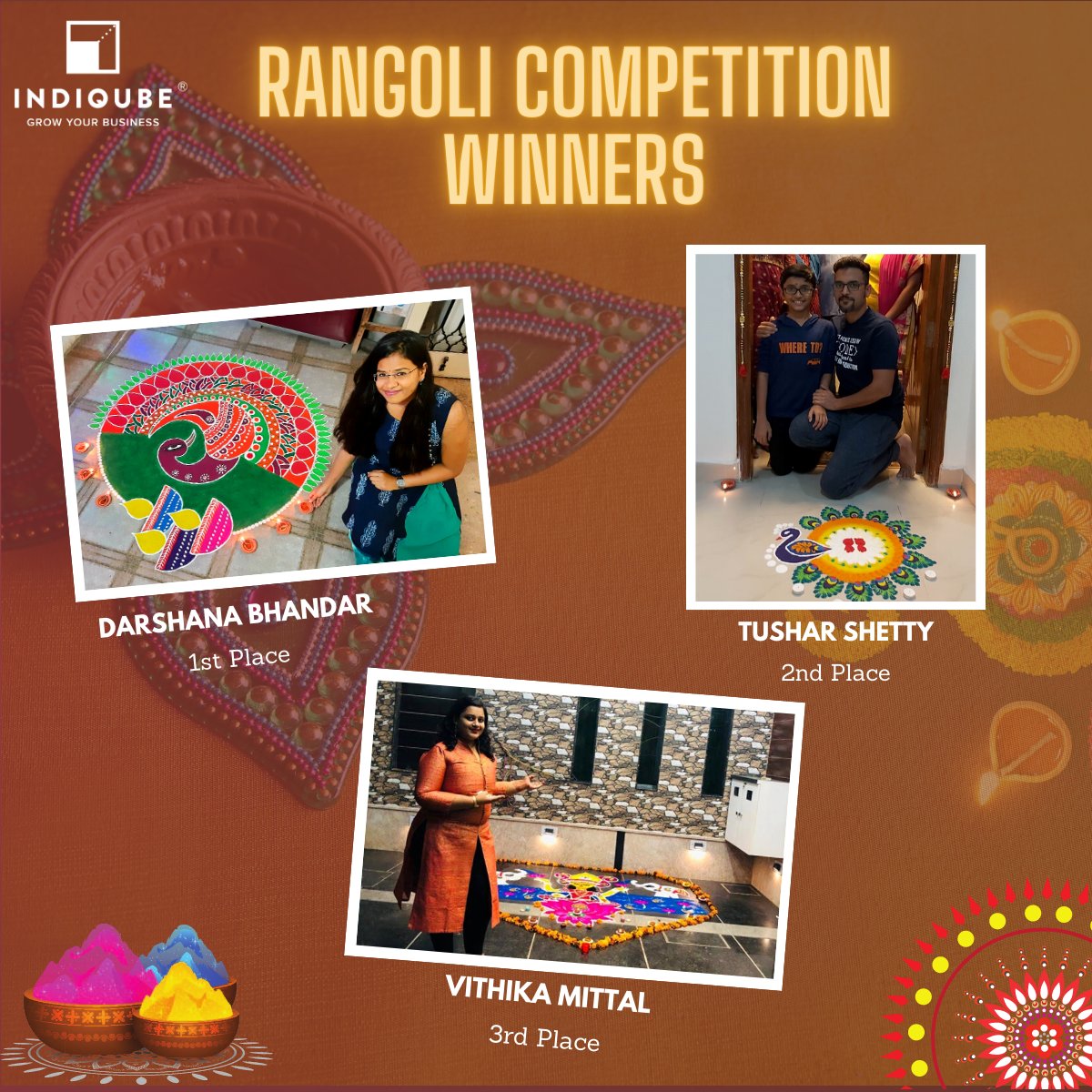The poster celebrating the Rangoli competition winners prominently features vivid details and a vibrant Indian theme. At the top of the poster, in large, glowing yellow capital letters, it says "RANGOLI COMPETITION WINNERS." Just below this, in the upper left corner, the text "Indicube" is displayed in white capital letters alongside their logo, and below this, it says "Grow Your Business." The background of the poster is a rich brownish color adorned with intricate Indian patterns. 

The winners are showcased with their names and positions:
1. **Darshana Bandar** - First Place, with a circular Rangoli design.
2. **Tushar Shetty** - Second Place, depicted as a young man with a vibrant bird design featuring green feathers.
3. **Vithika Mittal** - Third Place, presenting a heart-shaped Rangoli with colorful patterns inside.

Each individual has their photograph and design displayed on the poster, corresponding to their winning positions. The bottom left corner houses copper-colored bowls filled with glowing powders in magenta, yellow, and blue, adding to the festive, colorful atmosphere. The overall layout is visually balanced with thematic elements such as a star shape in the upper left and a circular pattern in the bottom right, enhancing the traditional Indian aesthetic.